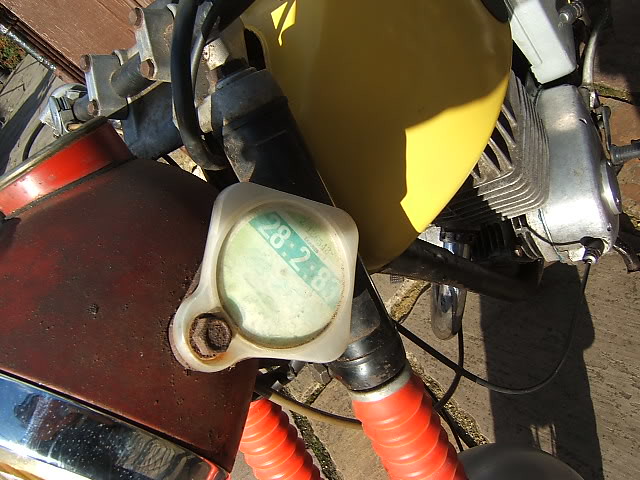This outdoor photograph captures a vintage, mechanized bicycle from an unusual angle. The bike appears weathered and aged, suggesting considerable use over time. Originally painted red, the bike's exterior now shows signs of wear, with patchy paint and darkened areas revealing its metal framework. Prominently featured on the left side is a metal spotlight, designed to provide illumination for nighttime riding, though this picture was taken during the day. Attached to the headlight with a hefty bolt is a faded white plastic piece, which bears a green label with the cryptic numbers "28..2..83". This numerical sequence remains a mystery. Visible behind the spotlight are black structural bars interwoven with red, accordion-like, tubular components that contribute to the bike's framework. Further back, a yellow plastic piece resembling an upside-down bowl encases the bike’s motor, hinting at its mechanical complexity.